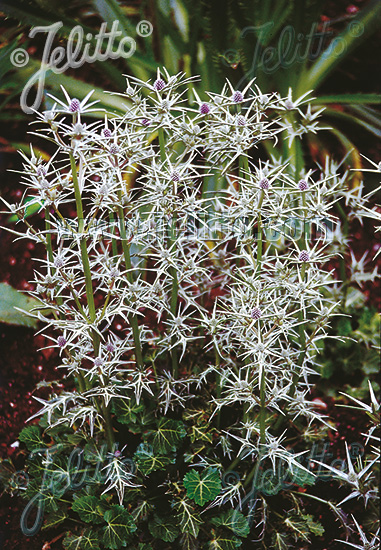In this high-definition close-up image, we see a prominent, spiky plant that seems to blend elements of a flowering bush and a porcupine. The plant features dense clusters of sharp, silverish-white petals creating a visually striking contrast against its green leaves and stem. Tiny white or yellow buds are scattered along the stems, resembling flowering bushes, while a central red berry-like element adds a pop of color at the heart of the plant. This vivid plant stands out in sharp focus, set against a blurred background that includes green palm tree-like structures with yellow-striped leaves and additional red berries on both the bottom right and left corners. In the top left corner, the photograph is marked with a white copyright symbol and the word 'Jelito' spelled J-E-L-I-T-T-O, which is mirrored as a faded logo in the top right corner. The image is suffused with various transparent copyright symbols, giving it a stock photo appearance while emphasizing the unique and potentially prickly texture of the plant.